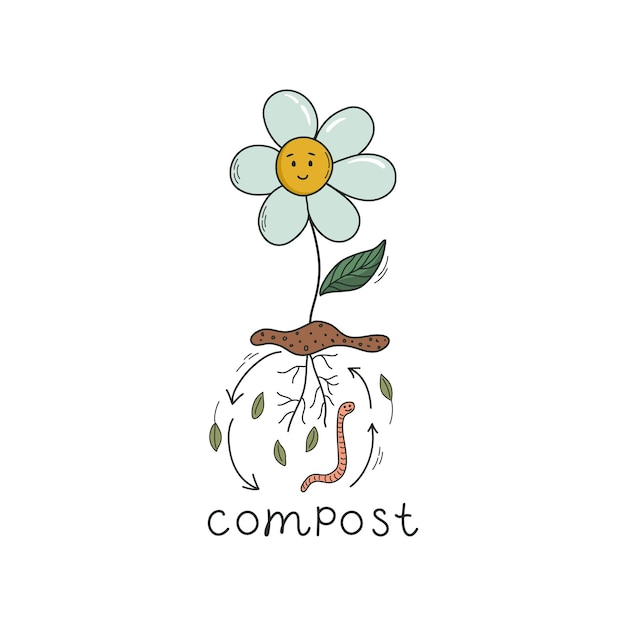This colorful cartoon illustration demonstrates the composting process in a simple and engaging way. The image features a cheerful daisy with a smiling yellow face and six white petals, growing from a thin, dirt-entwined stem with a single leaf. The flower is rooted in a small patch of soil, beneath which an animated scene unfolds: arrows move in a circular fashion around the roots, leaves, and a smiling, light brown-reddish worm shaped like an 'L.' These arrows highlight the cyclical nature of composting, emphasizing how organic material breaks down in the soil to nourish plants and support beneficial organisms. At the bottom of the image, the word "compost" is printed in clean, black, lowercase font, reinforcing the educational theme on a pristine white background.